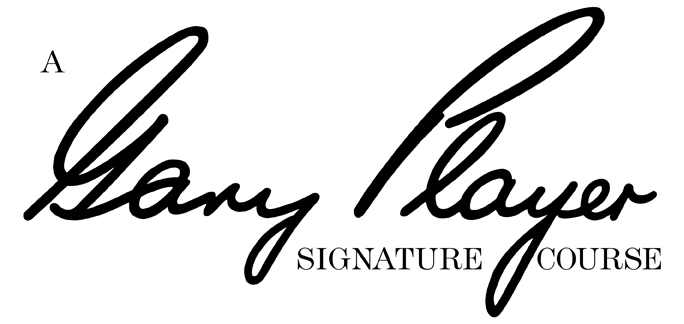The image depicts a logo on a white background featuring the signature of golfer Gary Player. The signature, written in bold, black, italic cursive, captures the elegant flow of Gary Player's handwriting. In the upper left corner of the image, there is a capital letter "A." Below and interwoven with the signature, the words "SIGNATURE COURSE" are prominently displayed in all caps, completing the logo. The black text on the white background highlights the prominence of the signature and the associated golf course brand that it represents.